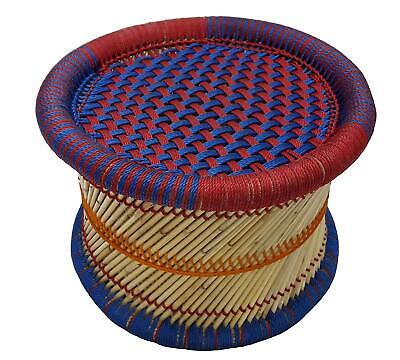This photograph showcases a uniquely designed object resembling the shape of a spool, potentially a seat or a footstool, characterized by intricate weaving and vibrant colors. The top part, which is the widest section, features a circular surface divided into four quadrants—two red and two purple. This surface exhibits an interlocking pattern created by red and blue lines, forming a striking weave.

Below the top, the central section narrows into a tube-like shape made from tan wicker material, accentuated by a ring of brown. This cylindrical middle part is adorned with sections of red and dark blue weaving, giving it a rich texture and depth. Furthermore, the upper and lower ends of each wicker strand are tied with small red ribbons, adding a delicate decorative touch.

The base of the object is a bit wider than the center but smaller than the top, contributing to its spool-like appearance. This base is primarily blue with dark red stripes interwoven throughout, along with touches of yellow. The meticulous craftsmanship and alternating color scheme make this piece both functional and aesthetically pleasing.